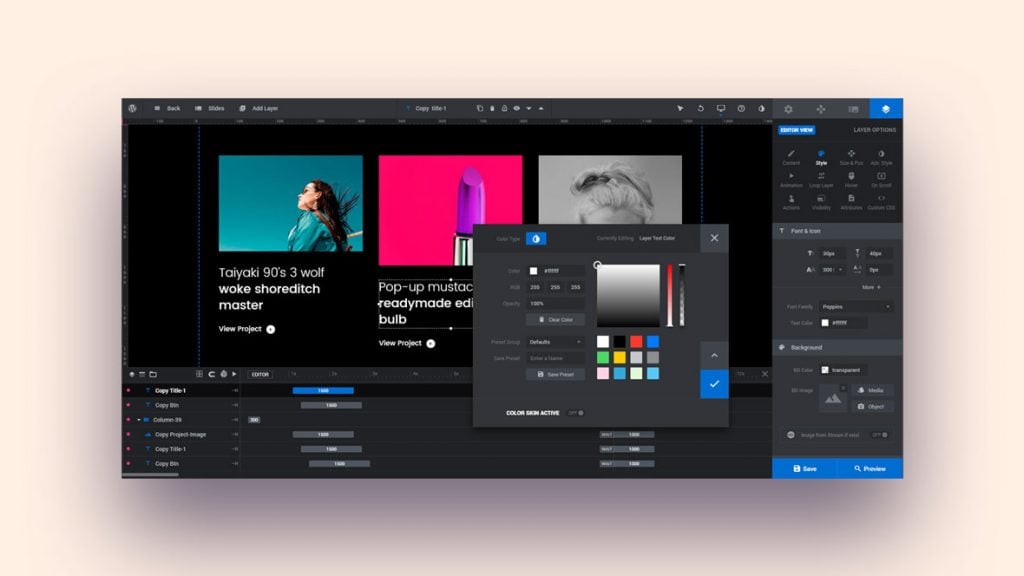The image showcases an intricate interface design with various colorful and interactive elements. On the top left, there's a section featuring options for background customization in either purple or pink, accompanied by icons for backslides, adding layers, and copying elements. The right side is populated with a diverse collection of icons and tools, including options for fonts, backgrounds, saving, and previewing the final design.

In the center-left portion of the interface, a prominent blue square stands out, accompanied by an assortment of descriptive keywords such as "long hair," "Taiyaki," "90s," "three wolf," "woke," "shore," "ditch," and "master." Immediately next to a vivid red square labeled as "lipstick," there's a pop-up indicating its presence. Just below, a gray square is visible, contributing to the neutral tones of the interface.

Moreover, a color selector tool is integrated, providing choices of white, black, red, blue, green, yellow, and purple. Below the color selector are six horizontal rows, featuring repetitive gray and blue gradients in the sequence: gray, gray, gray, gray, blue, blue. The detailed design of this interface reflects a blend of functional and aesthetic elements, aimed at providing a dynamic user experience.